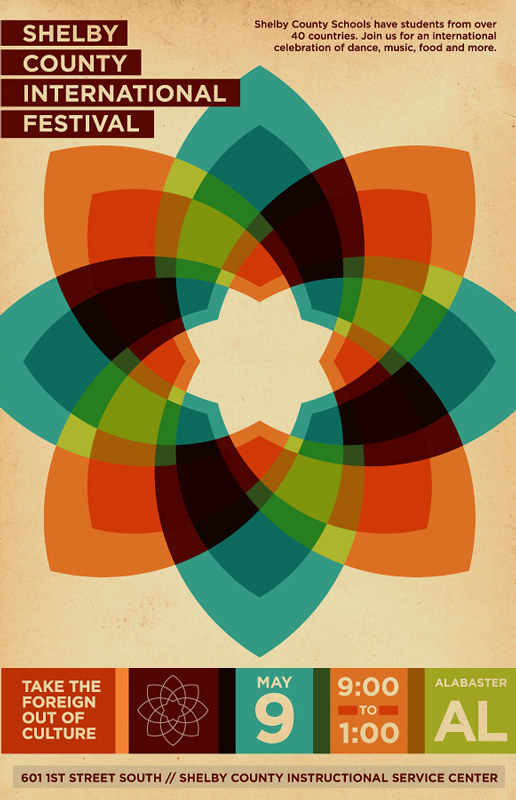The poster for the Shelby County International Festival features prominently in the top left corner with an inviting brown banner and translucent text, announcing the event. In the top right, the text emphasizes the vibrant diversity of Shelby County Schools, highlighting that students hail from over 40 countries. The poster invites the community to join a rich international celebration of dance, music, food, and more. Dominating the central area of the poster is an intricate, colorful geometric design that resembles a flower, comprised of overlapping shapes in a kaleidoscope of hues such as teal, orange, chartreuse, cream, red, green, yellow, and blue. Below this artistic display, the poster encourages participants to "take the foreign out of culture." Adjacent to this message, a similar geometric design indicates the event details: May 9th, 9 AM to 1 PM, at Alabaster, with the location specified as 601 First Street South, Shelby County Instructional Service Center. The background of the poster is a soothing tan or brown color, providing a warm backdrop for the vibrant festival announcement.